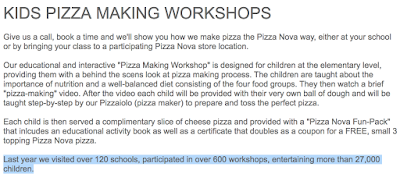"Kids Pizza Making Workshops by Pizzanova"

This promotional poster invites schools to Pizzanova’s Kids Pizza Making Workshops, which are designed for elementary-aged children. The invitation reads in gray, all-capital letters and encourages schools to give them a call to book a session. Participants can attend the workshop either at their school or at a participating Pizzanova store. 

The workshop is both educational and interactive, offering children a behind-the-scenes look at the pizza-making process, despite a small typo—'scenes' is misspelled as 'scens.' The children will learn about the importance of nutrition and maintaining a well-balanced diet consisting of the four food groups. The experience begins with a brief pizza-making video. Afterward, each child receives their own ball of dough and is taught step-by-step by a pizzaiola, or pizza maker, on how to prepare and toss the perfect pizza. Once the hands-on session is complete, each child enjoys a complimentary slice of cheese pizza and receives a Pizzanova fun pack. The fun pack includes an educational activity book and a certificate that doubles as a coupon for a free small pizza with three toppings.

The poster proudly highlights that last year, Pizzanova visited over 120 schools, conducted more than 600 workshops, and entertained over 27,000 children.